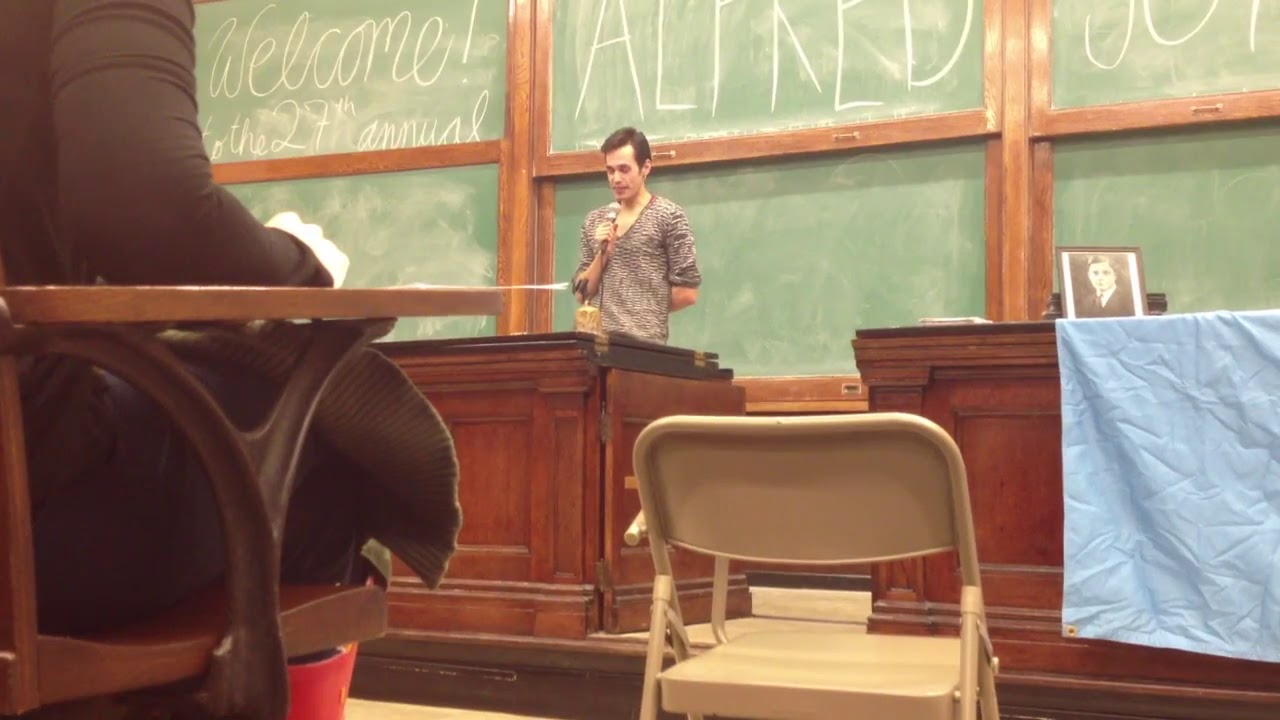The image captures a lecture or meeting scene set in a classroom or meeting space oriented in landscape format. Central to the photograph, slightly to the left, is a man around 35 years old, who appears to be giving a speech or lecture. He is wearing a grayish-beige v-neck shirt with black horizontal stripes, and his sleeves are pushed up to his elbows. The man is holding a microphone and looking down at a wooden podium, likely in the midst of his presentation. 

In the background, a large green chalkboard divided by wooden cross pieces spans the wall. Written in white chalk across the top, the board reads, "Welcome to the 27th Annual..." with some of the latter words cut off, including segments that spell out "A-L-I-N-E-D" and "joy." 

To the right of the speaker, a desk draped with a blue plastic tarp is visible, atop which sits a framed black-and-white vintage portrait of a man. In the foreground, a person in black attire is partially visible, seated at a desk on the left side, with only their partial arm and leg showing. Next to this desk is an empty beige folding chair. The setting combines elements of realism and photographic representationalism, creating a detailed context of a formal academic or commemorative event.